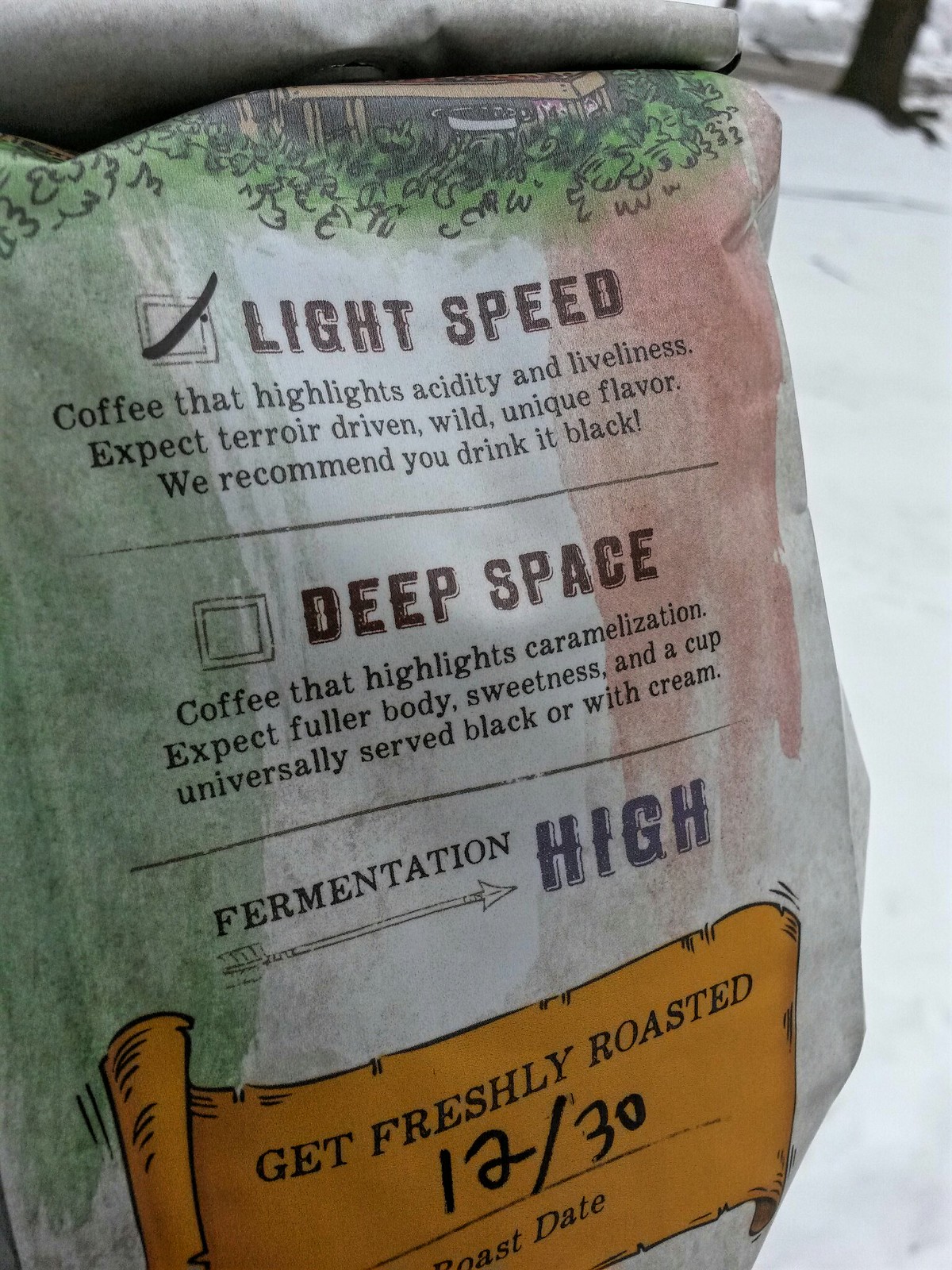The image displays a rectangular package of coffee with a primarily white background accented by green and brown hues. The top of the package is folded, and it features a design depicting green grass and possibly a coffee plantation. A brownish swath runs down one side of the package, contrasting with the green on the other side. 

Text on the package categorizes the coffee into three distinct types: "Light Speed," "Deep Space," and "Fermentation: HIGH." The "Light Speed" option, which is indicated as checked, highlights acidity and liveliness with a terroir-driven, wild, and unique flavor, recommended to be enjoyed black. The "Deep Space" option focuses on caramelization, offering a fuller body and sweetness, suitable to be served black or with cream. The "Fermentation: HIGH" option is also noted, although less detail is provided.

Additionally, an orange-colored scroll on the package indicates the coffee was freshly roasted on December 30th, with the date formatted as 12/30 (Roast Date). Positioned to the right side of the package, against a white ground possibly covered in snow, there's a tree trunk in black, adding to the serene setting. There are no visible people or hands, suggesting the package is placed on a surface, possibly in a room.